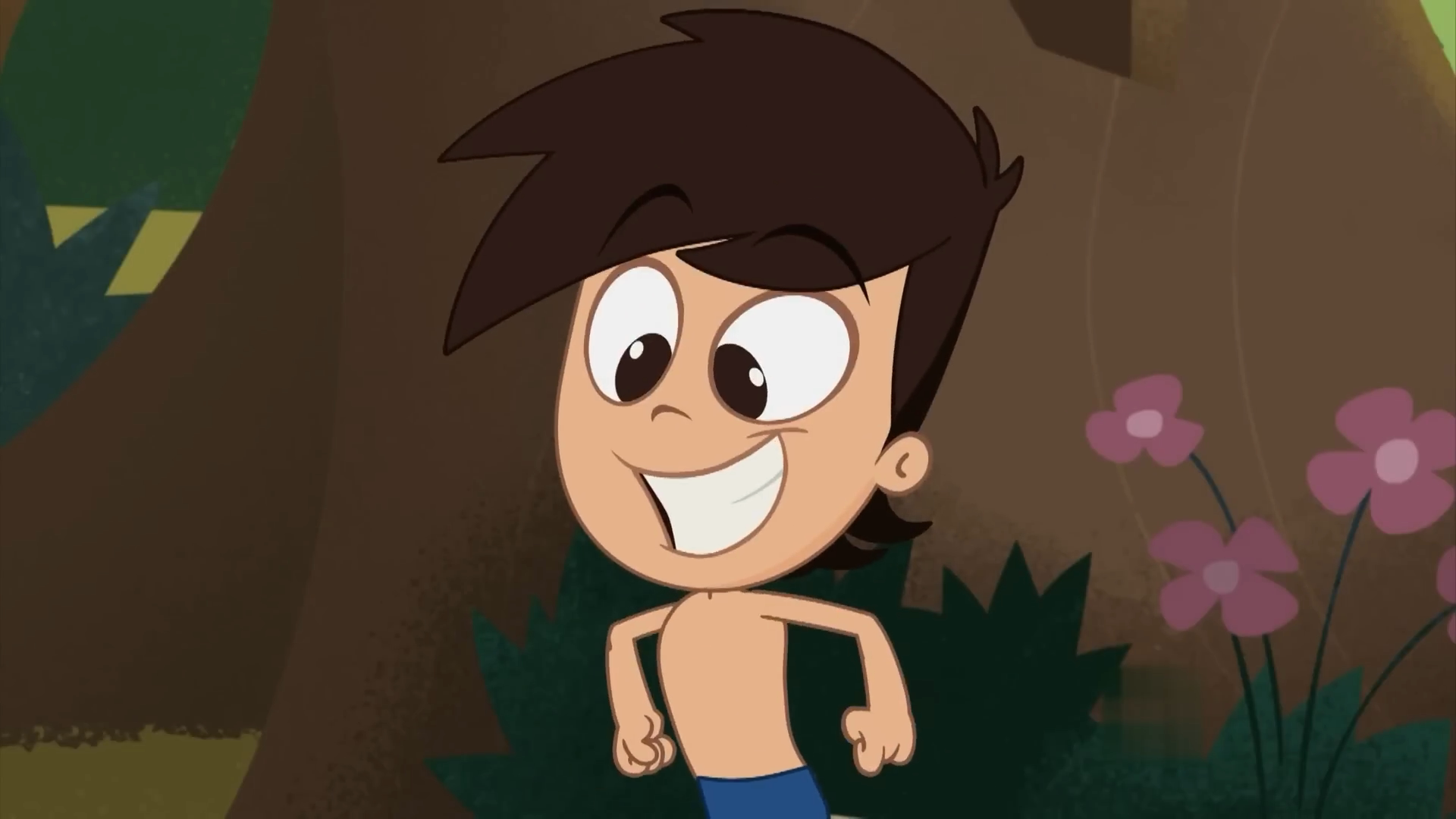This cartoon image features a white, shirtless boy with a giant, exaggerated head and big, oval eyes with black irises that give him a cross-eyed appearance. His thick, dark hair swoops over the top, resembling a mullet with big bangs. His equally exaggerated eyebrows are drawn prominently. He wears blue pants or shorts, though only the top part is visible as the image is cut off at the hips. Clenching his fists, the boy’s arms are held slightly out to his sides as he puffs out his chest. His face displays a large, sideways smile, revealing big white teeth. The background features a giant brown tree with purplish flowers in front of it, set against a brownish-greenish grass and greenish backdrop. No additional characters, text, or context are provided to explain the scene or the boy's cheerful expression.